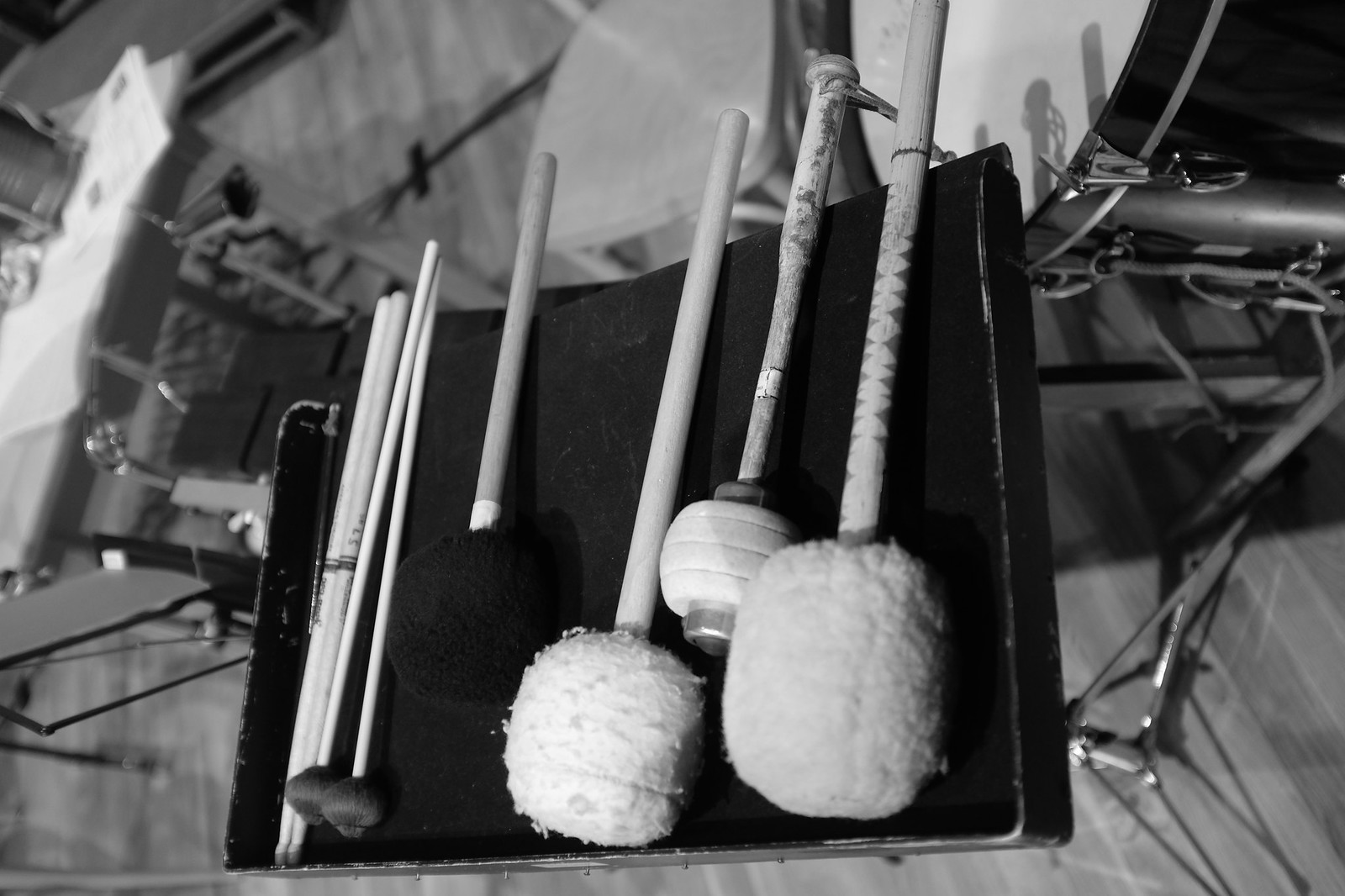This black-and-white photograph appears to have been taken from a slightly slanted bird's-eye view, and it captures a music room setting. Dominating the image is a black stand with a black tray, upon which various drumsticks and mallets are neatly arranged. Among these are two fuzzy mallets—one pair with white fuzz and another with black fuzz—each measuring about three inches long. There is also a cylindrical drumstick with grooves and a small metal disc at the top. Additionally, two straight, thin drumsticks lie to the left. Behind the stand, part of a drum kit is visible, with the white tops of the drums contrasting against the black drum bodies, which include a large tom or bass drum positioned on its side facing upward. To the left, there is a chair, and in the background, a blurred-out table with scattered papers and possibly another music stand can be seen. The room features lighter wood flooring, creating a stark contrast to the black elements in the image.